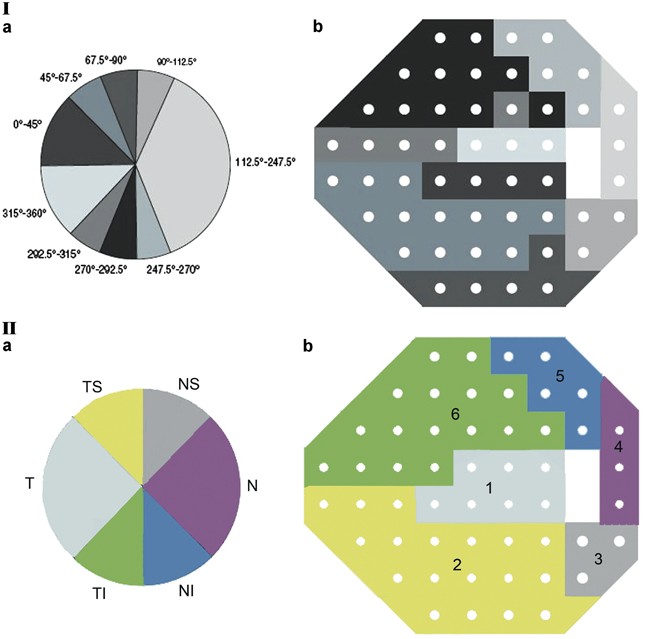The image is divided into two distinct sections: an upper and a lower. Each section contains two types of visuals on the left and right sides, respectively. In the upper left corner is a grayscale pie chart labeled "IA," featuring various shades from white to black. To its right is an irregular hexagon shape (referred to as "IB"), composed of a similar grayscale palette and dotted with white dots.

The lower section mirrors this setup. In the lower left corner (labeled "2A") is a pie chart displaying a more diverse range of colors—greens, blues, purples, yellows, alongside some grays. Adjacent to it, in the lower right corner (labeled "2B"), is another irregular hexagon shape. This one, like its upper counterpart, is also sprinkled with white dots, but it includes a broader spectrum of colors, matching those in the pie chart: green, blue, purple, yellow, and various shades of gray.

Both the pie charts and the hexagon shapes include specific labeling; the upper pie chart includes numerical divisions, while the lower pie chart shows labels like "tsnsnniit." The hexagons appear to be tagged with numbers corresponding to their color segments.